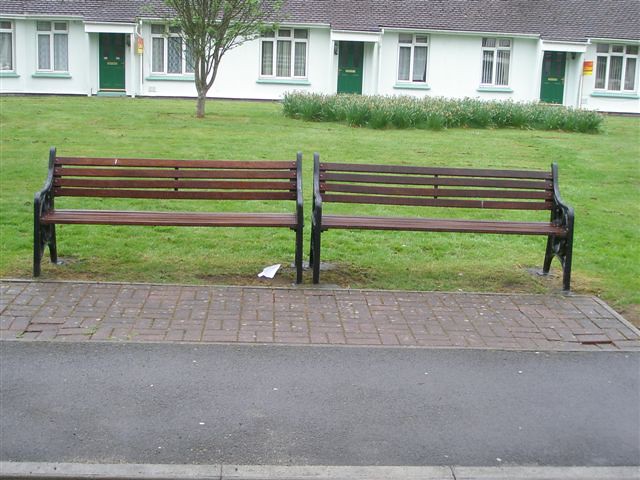This daytime photograph features two long, wooden park benches with thick black wrought iron arms and legs, positioned side by side on the edge of a vast, flat lawn. Immediately in front of the benches is a brick-paved sidewalk that alternates in a square pattern. Beyond the sidewalk, an asphalt road or path is partially visible. Behind the benches, the expansive grassy area includes a tree and a bed of flowers and shrubs to the right. Further back, there is a single-story white building with three green doors and several square windows uniformly spaced. The building appears to be part of a larger connected structure, possibly a row of apartments or an older motel. The grey slanted roof tops the building, adding a subtle contrast to the overall scene. The overcast sky suggests a calm, muted atmosphere, contrasting with the vibrant greenery and structured facade of the building.